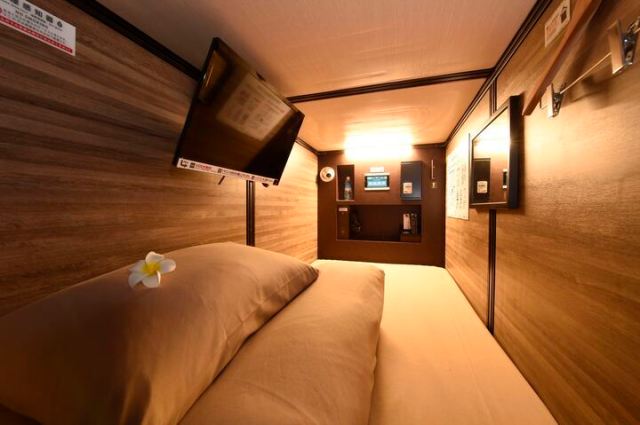This image depicts an exceptionally compact bedroom, possibly from a hotel or rented sleeping quarters, reminiscent of accommodations found in Japan or on trains. The room is entirely wood-paneled in a light to medium brown shade and lacks any windows, accentuating its confined space. Dominating the room is a twin-sized mattress that extends wall-to-wall, leaving no space on either side. On the bed, there are two pillows arranged with a small white flower featuring a yellow center delicately placed on top.

To the left of the bed, a large television is mounted on the wall, with a small white sign beneath it that likely contains safety information. The right wall holds another white sign written in an Asian language, indicating the room’s possible location or theme. Also on the right side is a rack with clips designed for hanging clothes, and what appears to be a shiny surface that could be a screen or possibly a built-in refrigerator or safe.

At the far end of the room, there are several built-in shelves and a bottle of water placed on one of them, providing minimal but functional storage options. The overall layout is reminiscent of a small, highly efficient sleeping space engineered for short-term stays or travel accommodations.